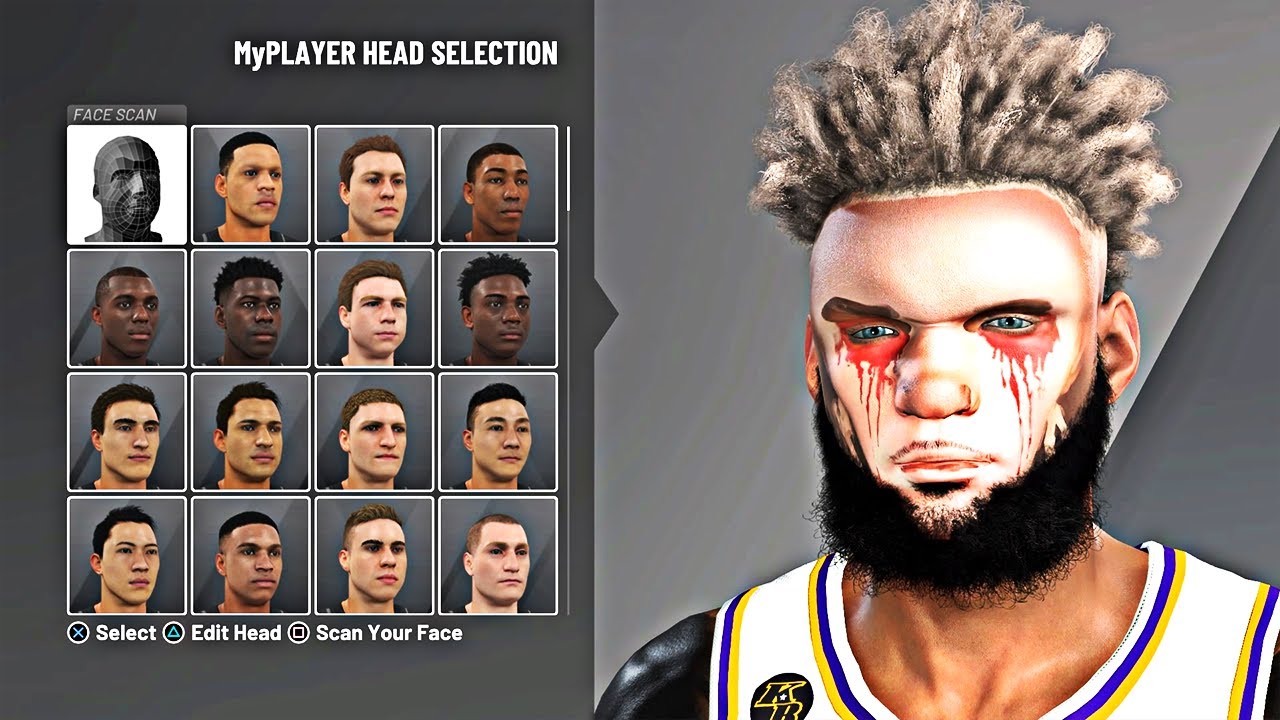The image appears to be a screenshot from a video game character selection menu, divided into two sections. On the left side, there is a box titled "My Player Head Selection, Face Scan," displaying 16 different head options that feature a variety of ethnic representations, including Caucasian, Asian, Hispanic, and African-American faces. The selection starts with a basic gray head model, presumably intended as a starting point for customization.

On the right side, a detailed character model of a basketball player is shown from the shoulders up. The player is wearing a white jersey featuring blue and yellow stripes and an emblem resembling a "K" accompanied by additional markings. The character sports a distinctive look with a dark black beard, pale facial skin contrasted by darker skin on the neck and ears, and compelling features such as blue eyes with streaks of blood flowing from them. His hair is styled in a unique combination of black-and-white dreads and an afro.